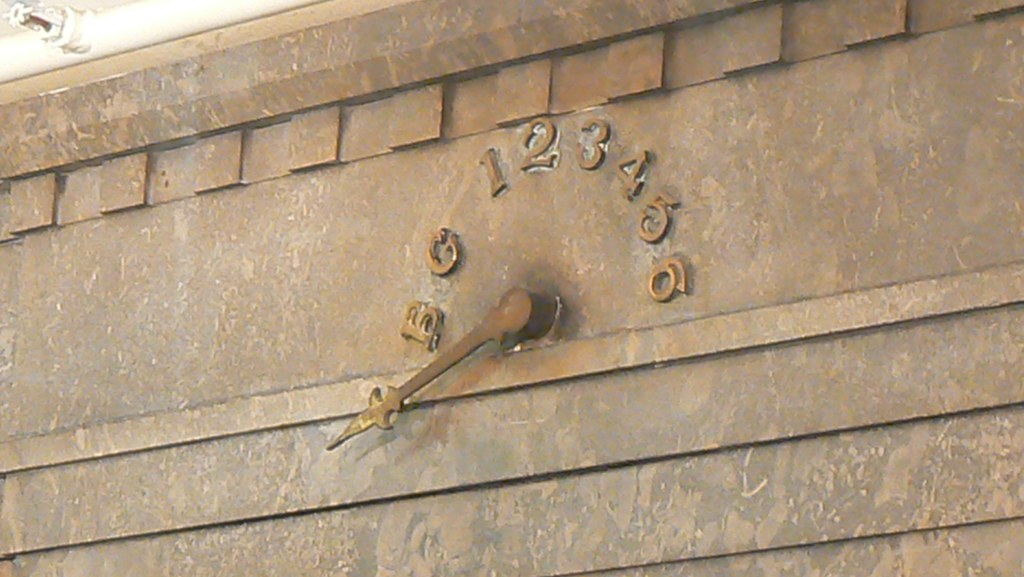This color photo captures a detailed, close-up view of an old-time elevator location marker on an outdoor stone facade. The wall is crafted from a mottled, light brown stone with a marbled, red, clay-like appearance. The stone texture appears somewhat dirty, and there are ornamental square accents just below a long arched strip. At the top of this ledge, numbers and letters—BG123456—are arranged in a semicircle, riveted into the stone, denoting basement, ground, and floor levels. An hour hand-like dial is prominently displayed, pointing out and almost rusty-looking, indicating the elevator's position. This detailed marker, devoid of the actual elevator in the frame, gives insight into the building's historical and architectural charm.